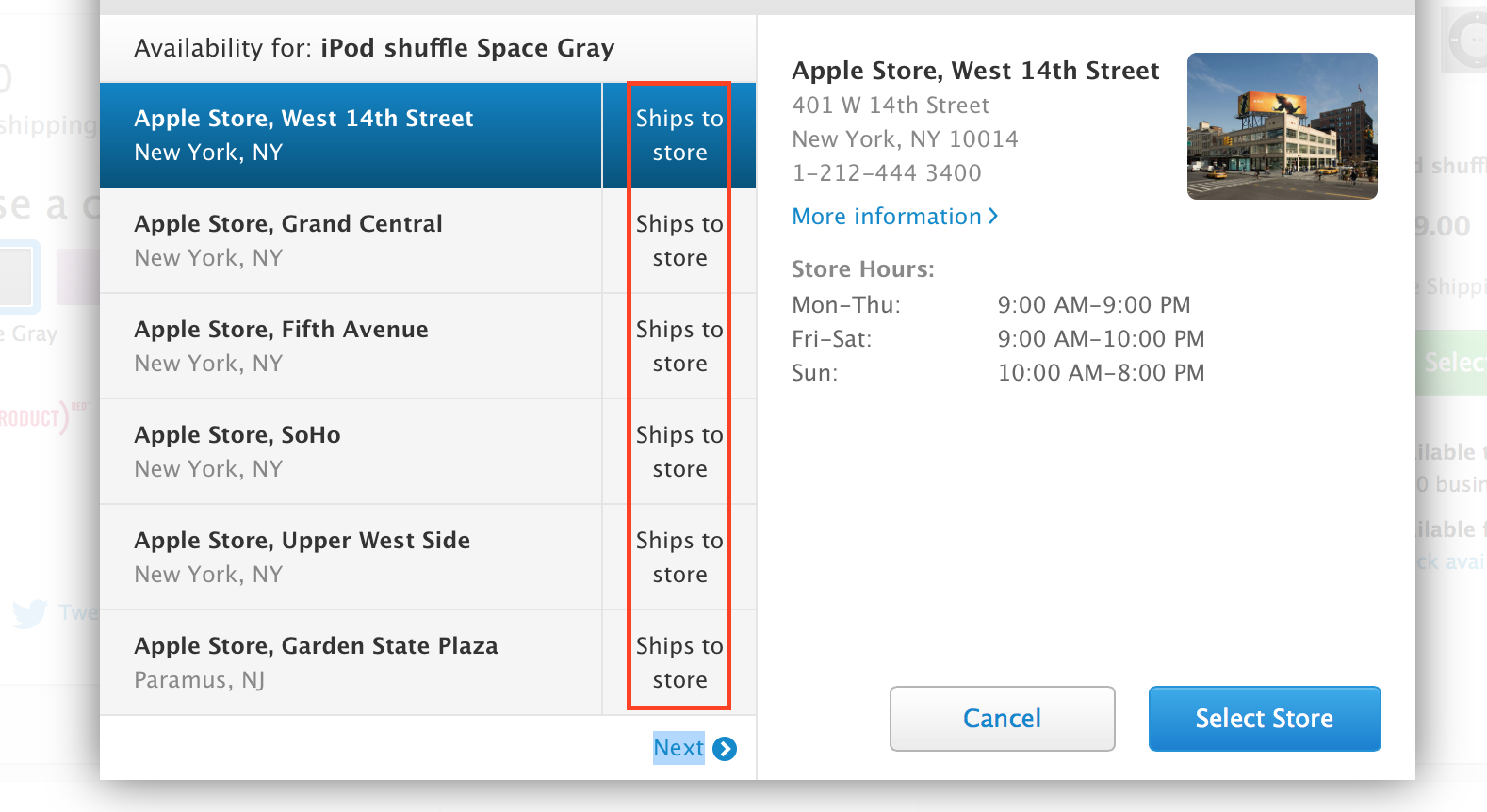The image is a screenshot of a computer interface, likely part of a website or a settings menu, which features a pop-up window displaying availability information for the iPod Shuffle in Space Grey. The interface primarily consists of black text on a white background, with greyed-out text on either side, indicating it may be overlaying another page. The pop-up window has a grey border with a slight shadow effect on the bottom and right edges, giving it a raised appearance.

At the top left of the window, the text reads "Availability for iPod Shuffle Space Grey." Below this heading, there is a column with six rows, each representing different locations for Apple Stores. The first row, highlighted in blue with white text, indicates "Apple Store, West 14th Street, New York, NY" and notes that the item "Ships to store." The subsequent rows list additional Apple Store locations: "Grand Central, New York," "Fifth Avenue, Soho," "Upper West Side, New York," and "Garden State Plaza, New York." All the locations have the "Ship to store" option highlighted by a red outline rectangle.

At the bottom of this section, there is a blue clickable box labeled "Next." The selected store, which appears to be the first one, displays additional details on the right side. These details include the store's full address, an image of the store showing a blue sky, a yellow sign above the roof, and a grey road in front of it. There are further details about the store's opening hours listed by days of the week: "Monday to Thursday," "Friday to Saturday," and "Sunday."

At the bottom of the pop-up window, there are two buttons: a "Cancel" button to the left, which is grey with blue text, and a "Select store" button to the right, featuring a blue background and grey text.